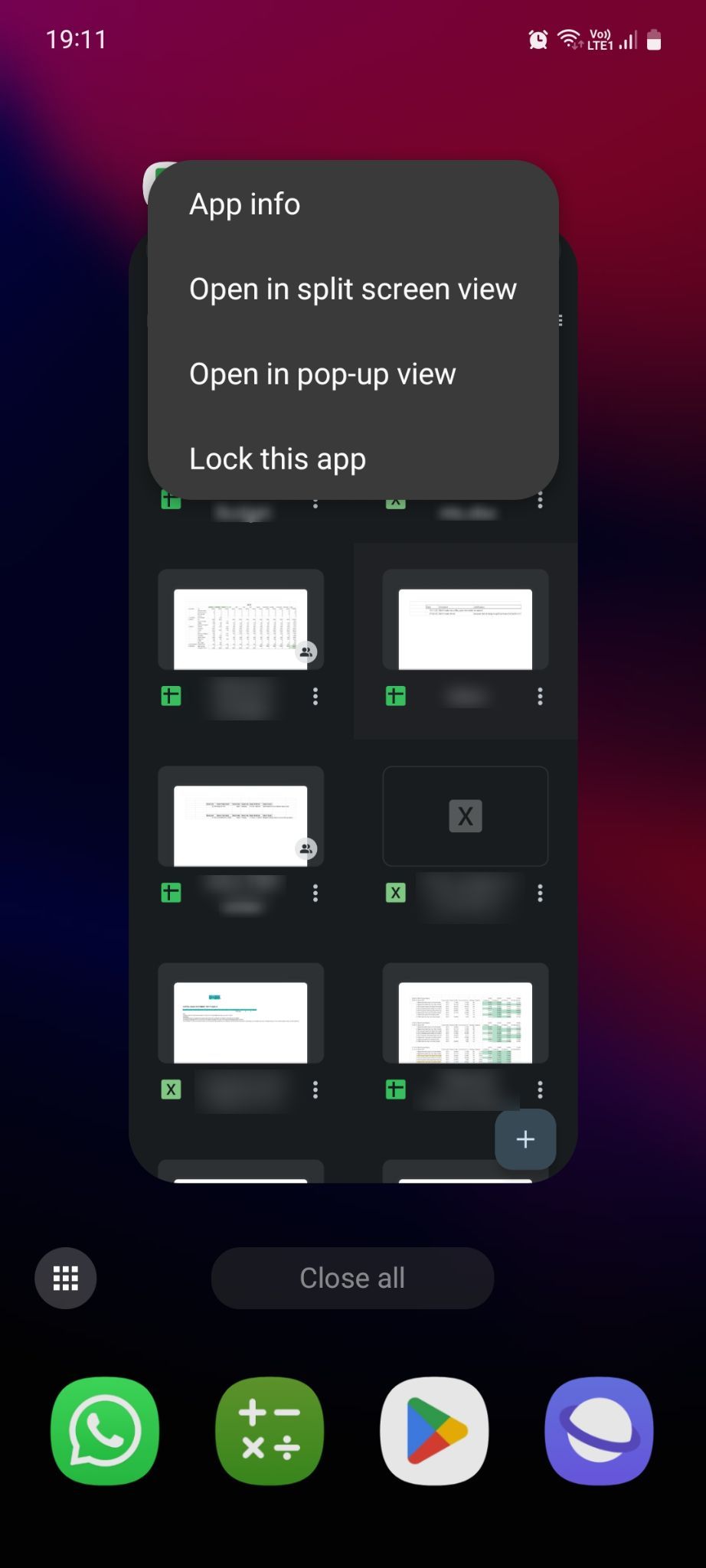This image is a screenshot taken from a cell phone, presented in a vertical, rectangular format. The background features a gradient, starting with a reddish hue at the top, transitioning to black towards the bottom and left side. In the upper left corner, the time is displayed as "19:11". On the opposite end, the upper right corner shows the battery and WiFi symbols, indicating signal strength and device power.

A pop-up message, located in the upper section of the image, includes a small gray rectangle with white text that lists several options: "App info," "Open in split-screen view," "Open in pop-up view," and "Lock this app." Below this pop-up, partially overlapped by it, there appears to be a section featuring miniaturized previews of open applications, displayed as small computer screens. These mini screens typically display text in black on white backgrounds, with some containing green areas.

Towards the bottom of the image, a large rectangular button is prominently labeled "Close all," suggesting a mechanism to close all open apps at once. Below this, at the very bottom of the screen, resides a row of app icons. From left to right, they include: 
1. A green icon with a white speech bubble and a telephone symbol.
2. A darker green icon with arithmetic symbols (plus, minus, multiplication, division).
3. A white icon containing a colorful triangle, reminiscent of the Google logo.
4. A purple icon depicting a white planet encircled by a purple ring.